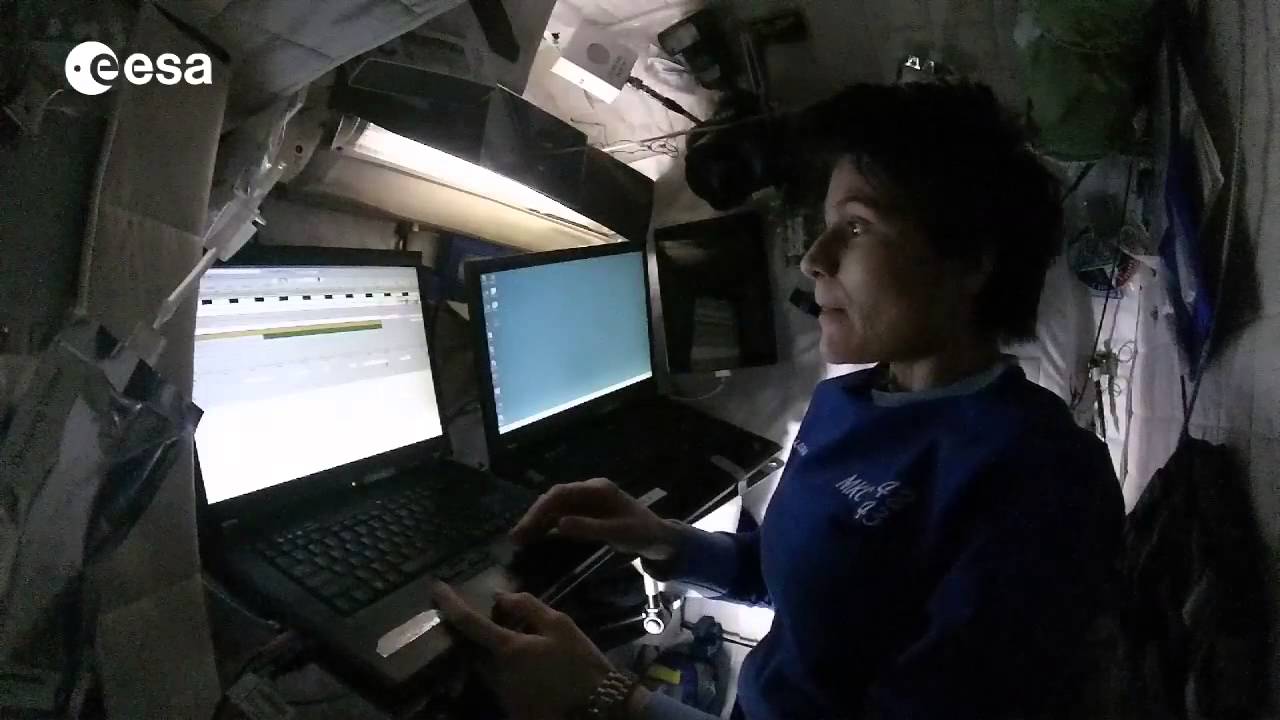The image depicts a woman with short brown hair wearing a blue long-sleeve shirt over a white shirt, sitting in a dimly lit, cluttered space that appears to be within a spacecraft or a similar environment. The setting is characterized by its irregular and floating objects, with no visible windows, enhancing the impression of zero gravity. The backdrop includes a sign with the acronym "EESA" on the upper left corner. She is fully focused on her work, her left wrist adorned with a silver watch. In front of her are two open laptops: the one on the left, displaying a white screen with various tabs, holds her attention, and she has both hands on its keyboard, suggesting she is actively engaged with it. The right laptop is on a blue startup screen. Although the exact nature of her work is unclear, it suggests she is performing navigational or technical tasks inside the spacecraft.